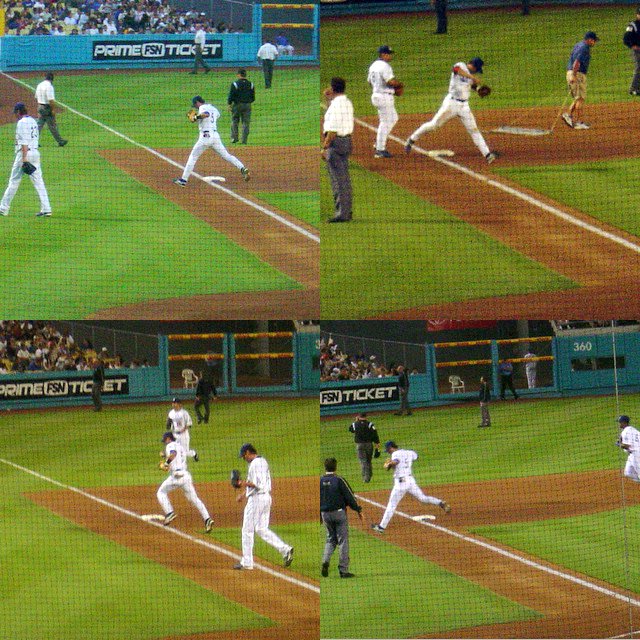This photograph is composed of four quadrants, each capturing a different moment from a baseball game. The scenes depict players dressed in white tops, white pants, and blue hats, actively engaged on the baseball diamond. One image features a player potentially running towards a base, with a glimpse of the crowded stadium seats behind him. Another quadrant shows a group of four men: two players, an umpire in black, and a groundskeeper raking the infield dirt. A third quadrant highlights three team members, with one appearing to be making a run to a base. The fourth image offers a different perspective of one of the previous actions. Surrounding the field are aqua-colored walls adorned with an advertisement that reads "Prime FSN Ticket" in white letters on a black background. The stands shown are filled with enthusiastic fans. A yellow-barred fence lines the outfield wall, adding to the ambiance of the lively baseball scene.